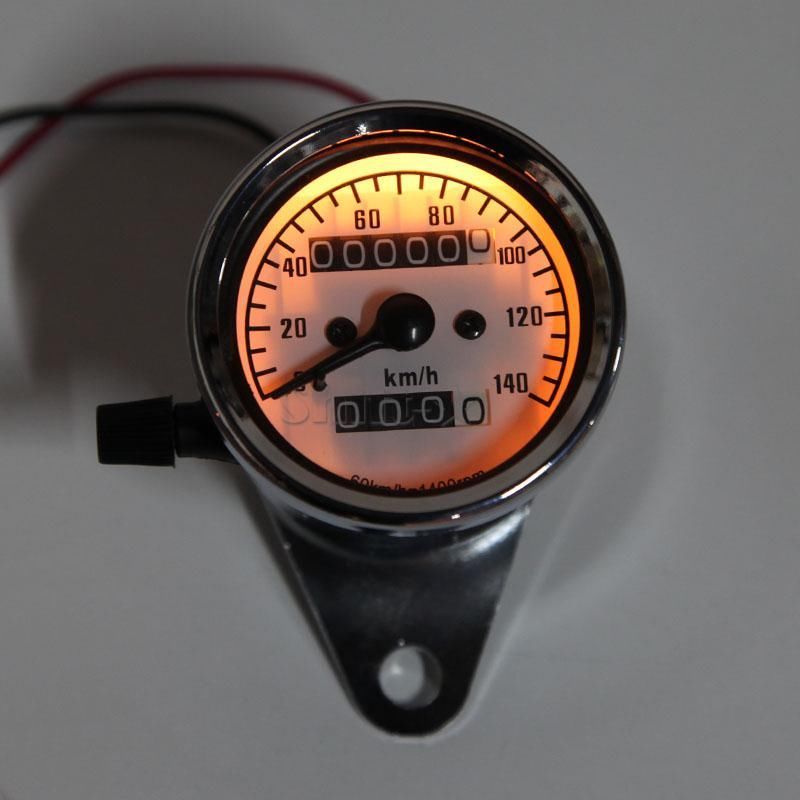This detailed photograph captures a dual-purpose gauge designed to measure both speed and mileage. Housed in a sleek stainless steel casing, the gauge features a clear display illuminated from behind or possibly the sides, enhancing visibility. The speedometer, marked in kilometers per hour, ranges from 0 to 140. The odometer, currently set at zero, sits prominently on the display, ready to log future journeys. A small trip meter is positioned at the bottom, which can be reset using a black knob located on the left side of the gauge. This knob can be pushed and turned to start a new trip count. A pair of wires protrude from the back of the device, indicating its electrical connectivity. The overall design combines functionality with a polished, modern aesthetic.